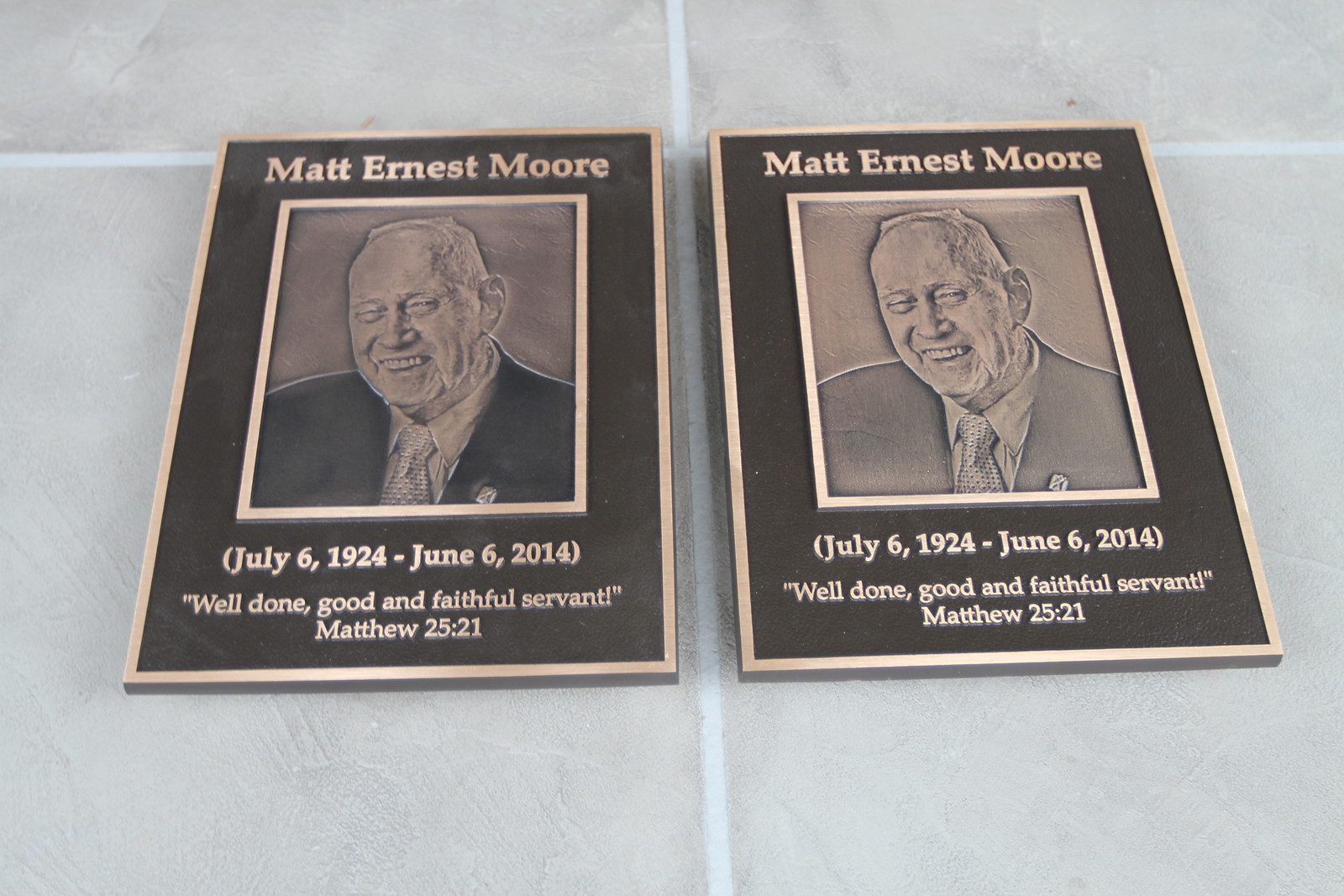This color photograph shows two bronze plaques with lighter gold borders placed next to each other on a light blue tile surface. Each plaque features an etching of an elderly man with a big smile, wearing a suit jacket, tie, and collared shirt. Both plaques are nearly identical, with the inscription at the top reading "Matt Ernest Moore" in white lettering. Below the image, it states "July 6, 1924 - June 6, 2004," followed by the quote "Well done, good and faithful servant!" and the biblical reference "Matthew 25:21." The only difference between the plaques is the slight variation in the shade of the man's suit jacket, likely due to lighting.